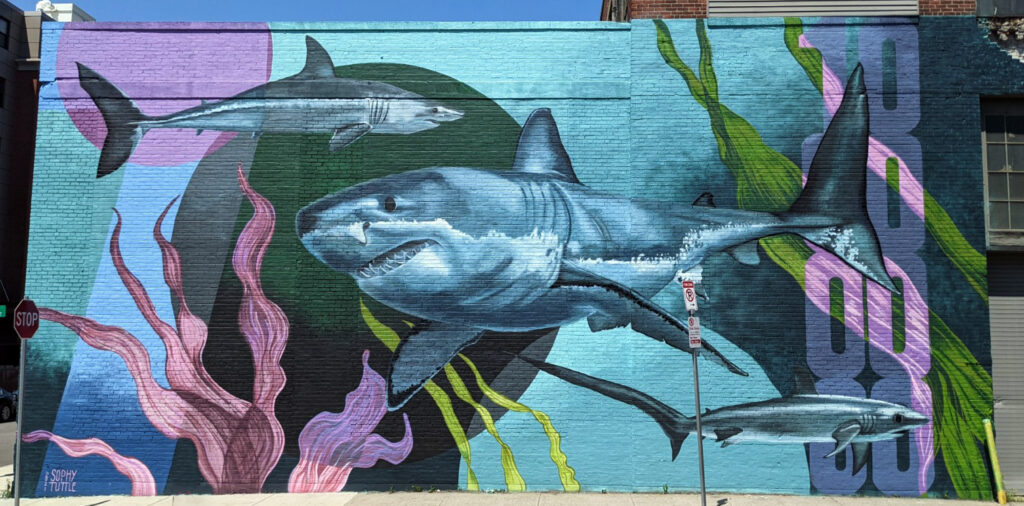The image is a detailed color photograph in landscape orientation, showcasing a vivid street mural painted on the side of a large brick building. This mural spans from top to bottom and left to right, with a small portion on the right side featuring an adjacent building with a window. The mural depicts an underwater scene filled with dynamic marine life and plant imagery. 

At the center of the mural, a prominent shark is illustrated with its nose pointing to the left and its tail towards the right. This central shark has a gray upper body, dorsal fin, and a white underbelly. Above this central figure, another smaller shark with an elongated nose is depicted swimming in the opposite direction, with its nose to the right and tail to the left.

Adding to the complexity of the scene, a third, much smaller shark with a longer tail and shorter snout is positioned at the bottom right of the mural, swimming towards the right. The mural features vibrant aquatic plant life, including wavy pink and purple seaweed on the bottom left and light yellow grasses rising from the bottom.

Two distinct circular shapes add a stylistic element: a smaller, semi-transparent pink circle in the upper left and a larger dark green circle to the left of the center, behind the sharks. Additionally, the number "0010" appears in stacked, semi-transparent purple color on the right side of the mural. Sea kelp and seagrass weave throughout the scene, creating a sense of movement and depth within this hand-painted, representational mural.